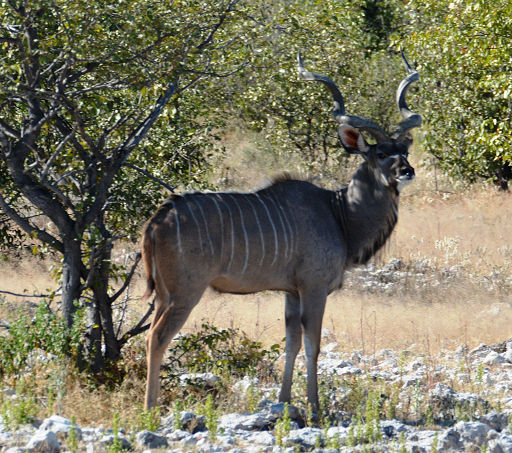In this square outdoor photograph, a deer is prominently featured in the center, set against a forested background. The deer, brown in color with white vertical stripes along its back, stands gracefully on skinny legs amidst a rocky, weedy area. Its two large, curved antlers rise above the head, which is supported by a long neck. The deer is facing to the right side of the image but has its head slightly turned towards the viewer, with its big ears perked up, giving a sense of alertness. 

Surrounding the deer is a mix of natural elements: there are rocks of a sand-like tan color, patches of green grass and weeds sprouting up between the rocks, and a cloud of dirt suggesting recent movement. A tree with sparse, thorny branches is directly behind the deer, and additional trees with more foliage appear in the background, extending upwards and partially frame the scene. The floor of the clearing is dotted with stones and covered in brown dirt, resembling a nature trail that weaves through the area. The setting conveys a tranquil yet dynamic wilderness scene, highlighting both the beauty of the deer and its natural habitat.